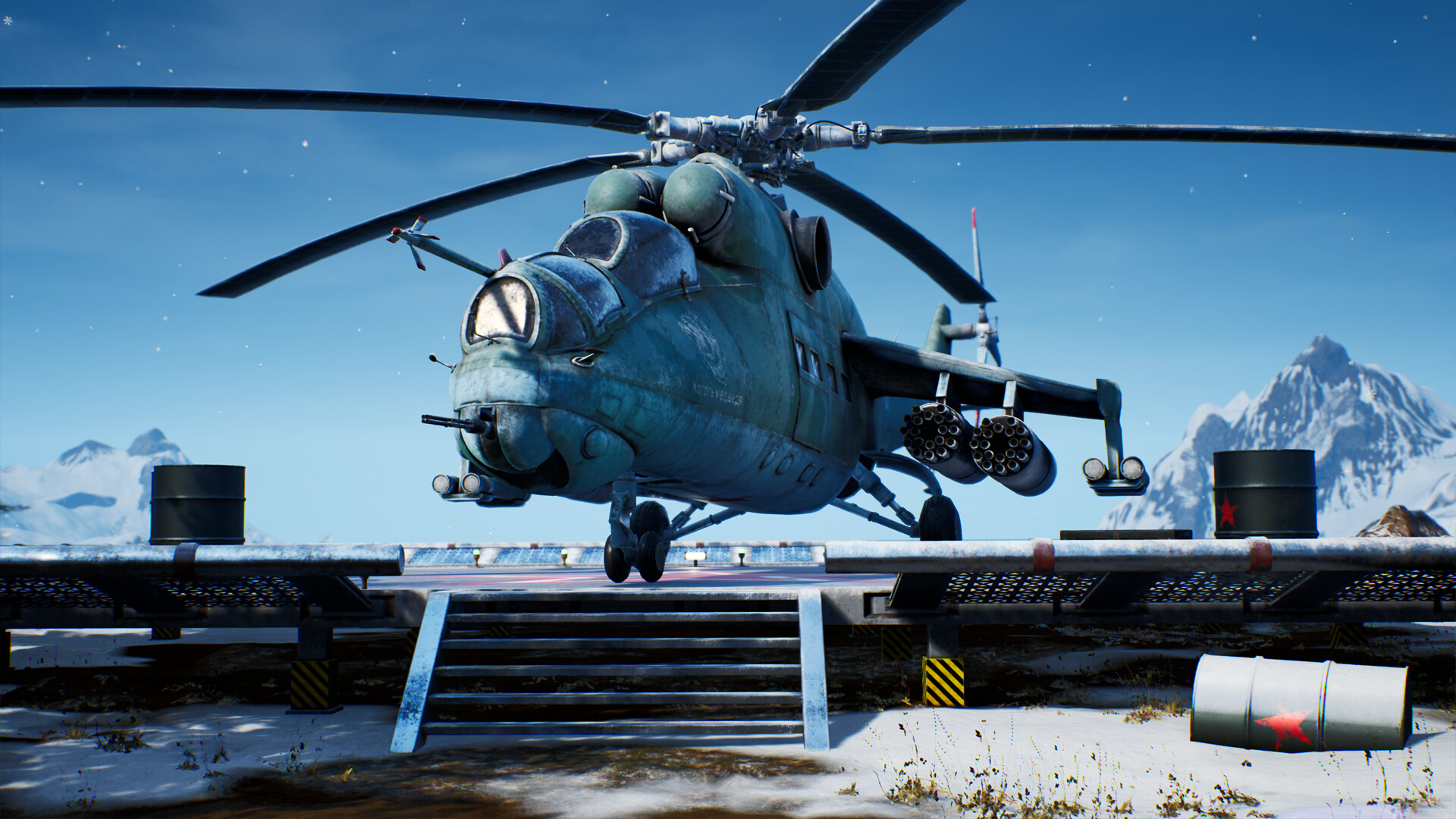The image is an outdoor screenshot from a video game, depicting a military-type helicopter with a grayish color scheme. The helicopter is either taking off or landing on a helipad, which is accessed by about six steps. The scene is set during the daytime, under a clear blue sky with shadows cast on the ground, adding to the bluish-gray aesthetic. Surrounding the helipad, the ground is covered in snow, and barrels and gas cans—both gray and black—are scattered around. Majestic snow-covered mountains rise in the background, enhancing the sense of a cold, remote location. The helicopter is armed with machine guns and missiles, suggesting it's ready for combat operations.